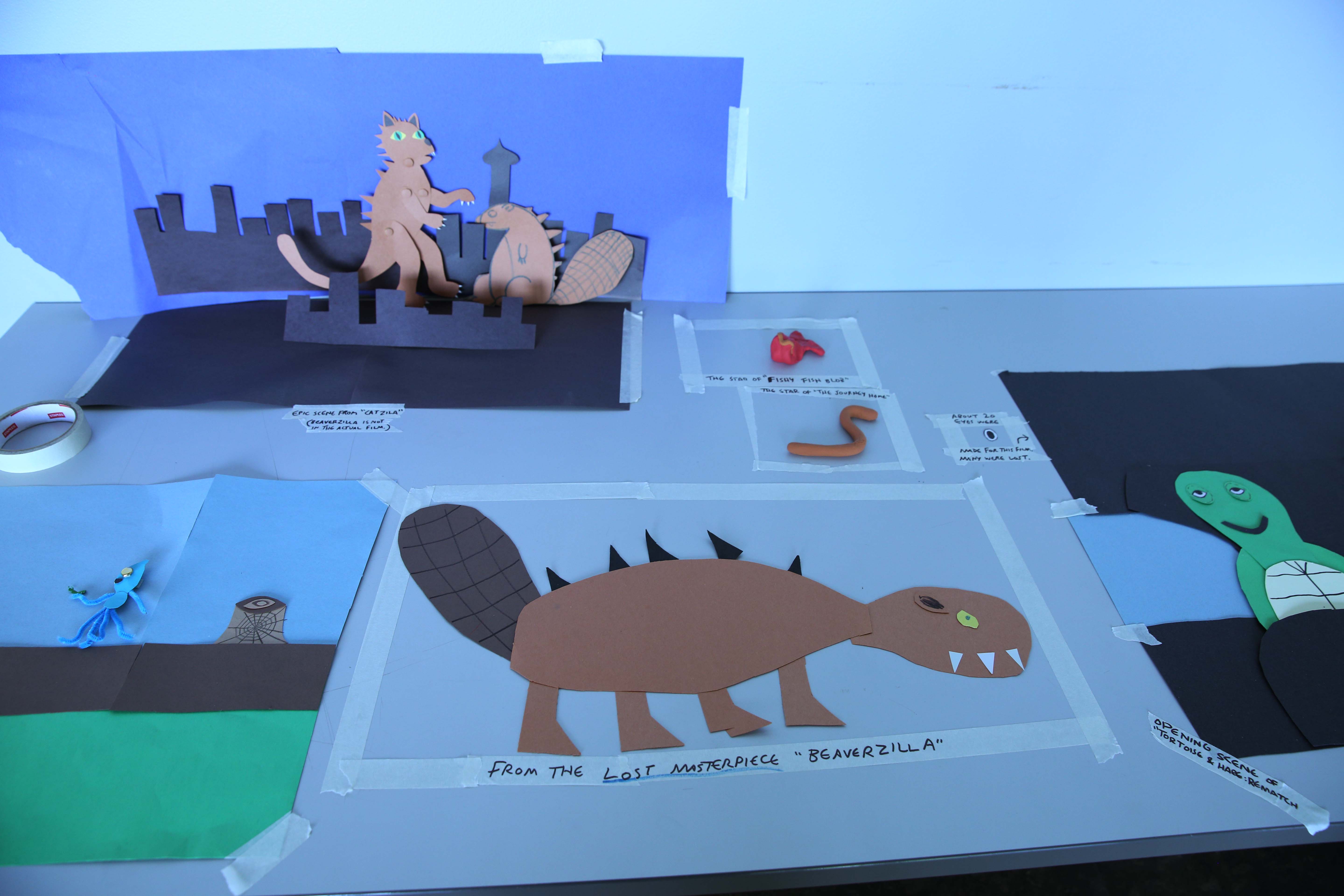The image depicts a detailed paper collage of children's artwork, spread out on a white surface with a white wall in the background. Central to the scene is a fierce-looking brown beaver, labeled "From the Lost Masterpiece, Beaverzilla," featuring sharp triangular spikes on its back, white fangs, and a dark brown tail. To the right of the beaver is a green turtle set against a dark background. Above Beaverzilla, a city skyline cut from black construction paper is set against a blue backdrop, appearing to host a battle between Beaverzilla and a large, cat-like creature. On the left side of the table, there is a roll of masking tape. The arrangement also includes smaller figures, such as a blue animal on a scene depicting a blue sky, tree stump, road, and green grass. The art is meticulously crafted from various colored pieces of construction paper, showcasing an imaginative and playful display of different characters and scenes.